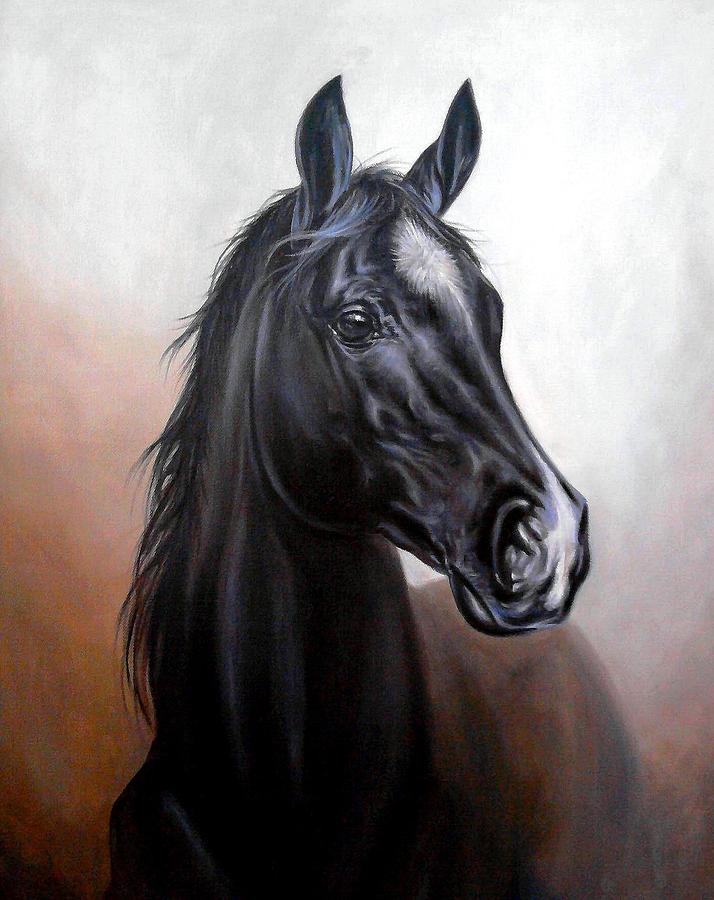This artwork depicts a highly detailed painting of a sleek black horse shown from the shoulders up. The horse's face is intricately rendered, showcasing expressive black eyes, alert and erect ears, and a nose with a distinctive white marking that extends up to its forehead. The mane is long and black, adding to the elegance of the animal. The background features an ombre effect, transitioning from a textured white at the top to soft bronzy browns towards the bottom, giving the impression of light and shadow play. The horse stands out vividly against this serene backdrop. Notably, the horse is bare, without any saddles or bridles, enhancing its wild and majestic appearance.